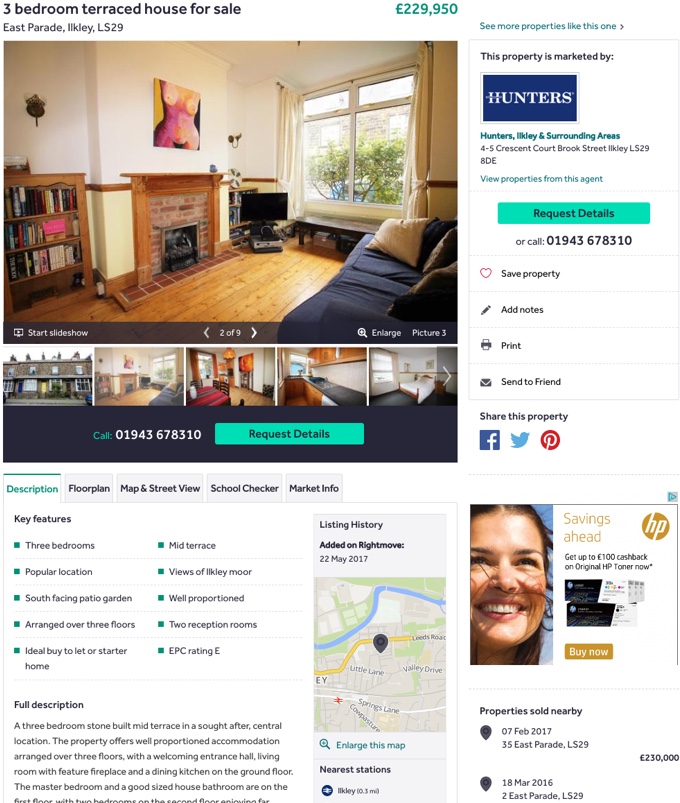**Detailed Caption:**

This vertical rectangle image showcases a real estate website or app interface designed for listing and browsing homes. At the very top of the image, there is a prominent heading that reads, "Three Bedroom Terraced House for Sale, East Parade, likely LS29," with an asking price of £229,950 clearly displayed.

Immediately below the heading, there is a main image of a cozy living room. This space features a central fireplace with an elegant mantle, flanked by two wall sconces. Above the fireplace hangs a picture of a naked woman, adding a touch of art to the room. To the left of the fireplace, there is a brown bookcase filled with books, contributing to the room's warm ambiance. On the right side of the fireplace, a television or monitor is placed on the ground. Additionally, a large window with curtains running the full length of the window adds natural light to the area. Adjacent to the window is a comfortable blue couch adorned with a couple of pillows. The upper part of the walls is painted white, while the lower section features a creamy yellow hue, creating a pleasant contrast.

Beneath the main image, there is a slideshow navigation bar indicating that this is image 2 of 9. Users can navigate through the images using the left and right arrows on either side. There is also an option to enlarge the current image, with a small indicator for picture number 3.

Further down, the interface shows five smaller thumbnail images of the property, each separated by white borders. At the far right of the thumbnails, there is an arrow for browsing additional images.